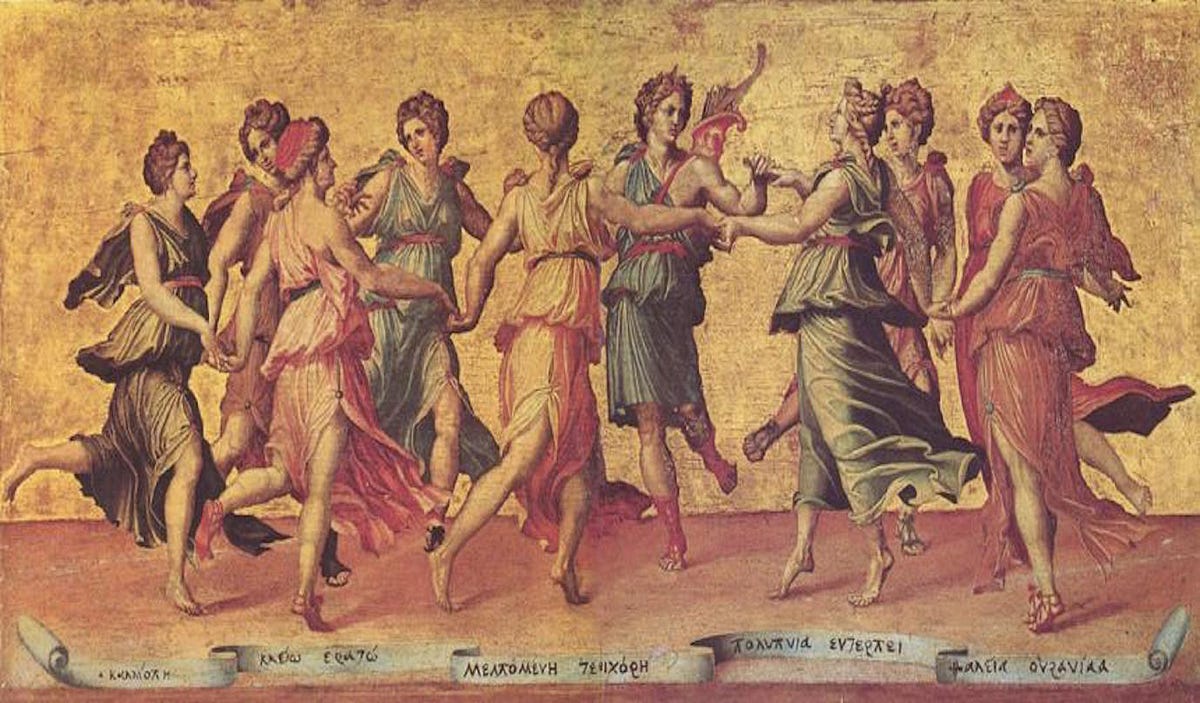This image is a faded, yellowed painting likely created during the Renaissance period, inspired by ancient Greek or Roman times. It portrays ten women dancing in a circle, holding hands as they celebrate. Each woman is adorned in a flowing robe with varying colors: black, brown, pink, blue, yellow, dark blue, green, another pink, red, and orange. Most wear red sashes around their waists, except for two with black sashes and one with a blue sash. The background resembles aged paper, and the women appear to be dancing on an indistinct ground. At the bottom of the image, a scroll with five sections unfurls, displaying text that is difficult to read, possibly written in an ancient or obscure language. The overall tone of the artwork is tarnished and ancient, suggesting it could benefit from restoration.